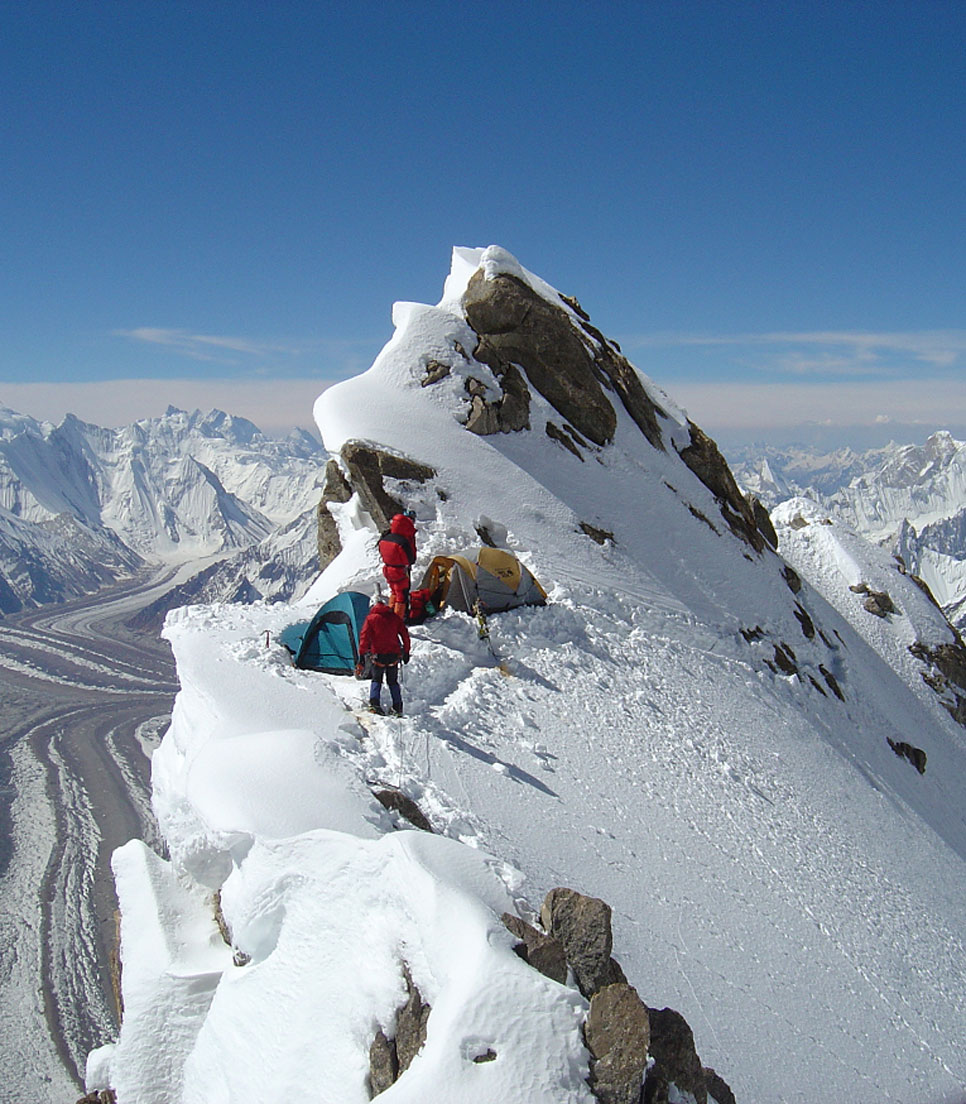The image captures a stunning scene of two mountain climbers near the top of a snow-covered peak. The climbers, clad in red jackets, are positioned just below the mountain's rocky summit, which is sprinkled with snow. The climber standing slightly higher wears a puffier red jacket with black shoulders and red pants, while the lower climber sports a regular red jacket and blue pants. Two tents are set up on the mountain—a turquoise and a yellow-and-gray one. The mountain is heavily blanketed in snow, with rocky patches peeking through. A network of tracks can be seen leading up the right side, and a road is visible on the left, hinting at civilization below. Beyond the immediate peak, an expanse of snow-capped mountains stretches into the distance, under a mostly clear blue sky adorned with a few wispy clouds. The sun illuminates the scene gently, enhancing the grandeur of the landscape.